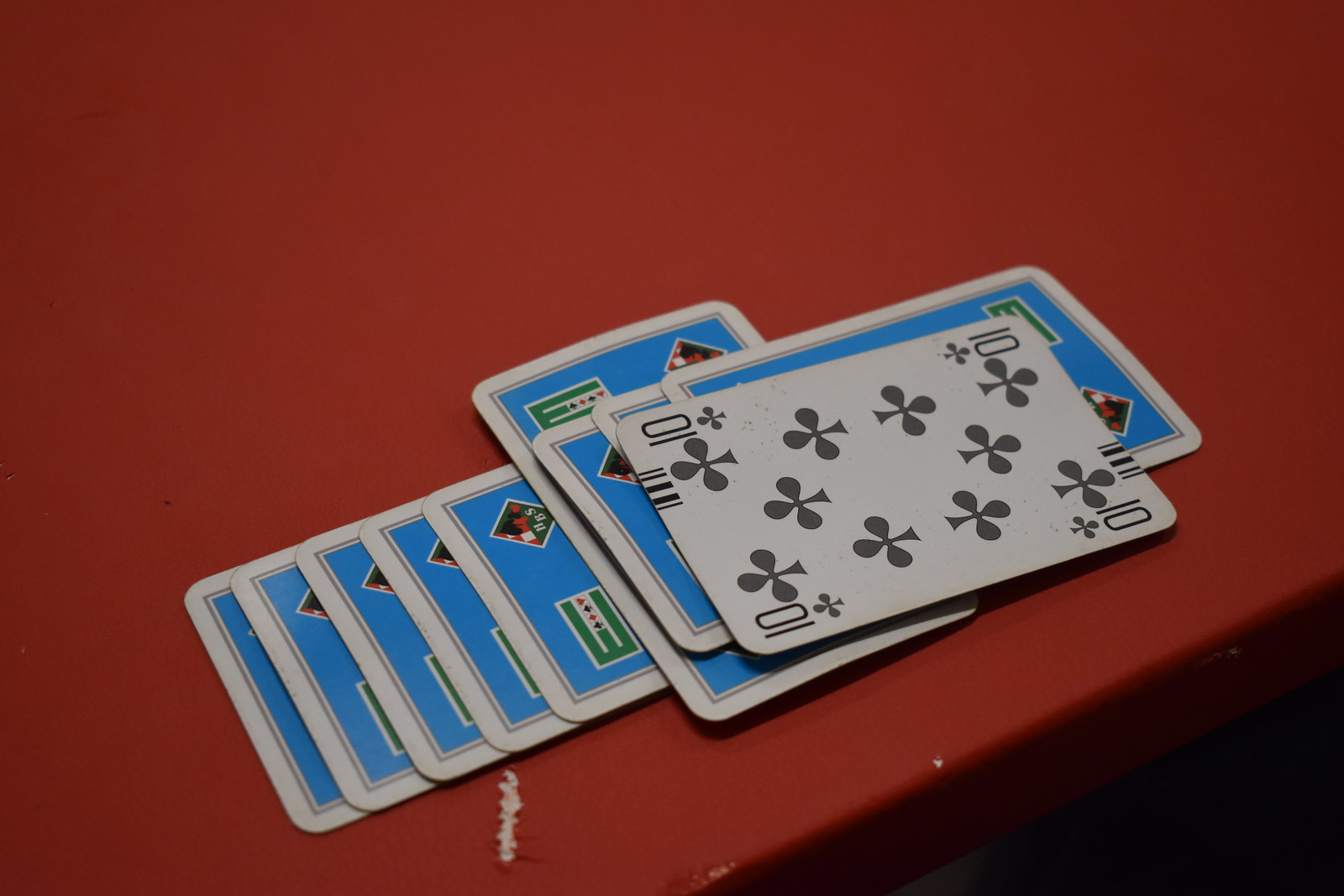A semi-stack of eight or nine playing cards is spread on the edge of a red table, prominently positioned in the lower right corner of the photograph. The cards predominantly face down revealing their blue backs, each adorned with intricate designs including what appears to be a miniature card and the logo of the card maker. Among them, the 10 of clubs is the sole card displayed face up, while another card in the middle of the line is oriented sideways. The vibrant red table exhibits distinct features, including a noticeable white scratch in its lower center. This arrangement gives the impression of a card game mid-play or simply a display of the deck's aesthetically pleasing backs.